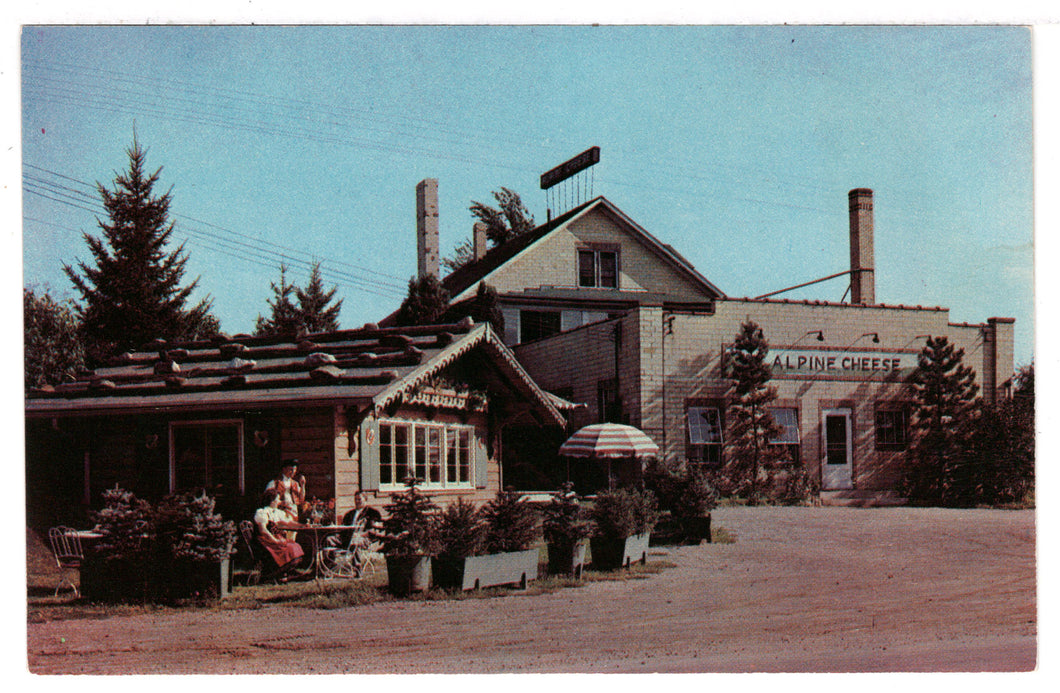The photograph depicts an old, faded image of a cheese factory or store with a prominent, white sign reading "Alpine Cheese." The main building, constructed from grey or white brick, features a central door flanked by tilted-open windows—two on the left and one on the right, alongside a tree. Above the door hangs a sign illuminated by three lamps. A thin chimney extends from the top right of the building. In the background, thin pine trees and power lines stretch horizontally across the sky. To the left and forefront of the factory, there is a single-story cottage with a pointed roof, blue shutters, and ornamental roof edging. This cottage's yard is adorned with several planters, and a large striped sun umbrella shades a table where two people, dressed in what appears to be Bavarian-style clothing, are seated. The scene includes additional tables, creating a welcoming outdoor dining area, suggesting that the building might also function as a restaurant where visitors can enjoy cheese and wine.